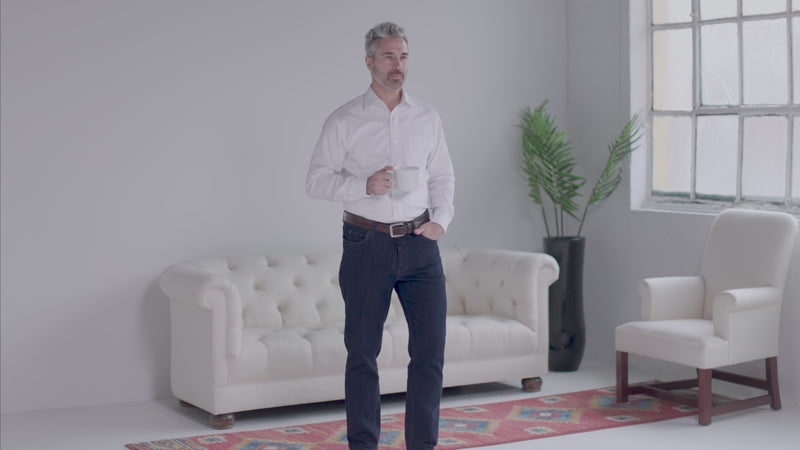In this image, a distinguished older Caucasian man with gray, salt-and-pepper hair, a mustache, and a neatly trimmed goatee stands in the center of a pristine living room. He is dressed in a white button-down dress shirt, tucked into dark blue denim jeans secured by a brown belt. One hand rests casually in his jean pocket while the other clutches a white coffee mug.

The room around him exudes a minimalist elegance. Directly behind him is a tufted white leather couch with rolled arms, flanked by a tall black vase holding several palm fronds. To the right of the couch, a cozy white fabric chair with wooden legs adds to the seating arrangement. The floor is partially covered by a white rug featuring a triangle pattern shooting from the center. A section of closed, rectangular windows on the right side of the room hints at the natural light that subtly illuminates the space. Every element in the room, aside from the black vase, plants, and rug, adheres to an all-white theme, creating a stark, modern aesthetic.